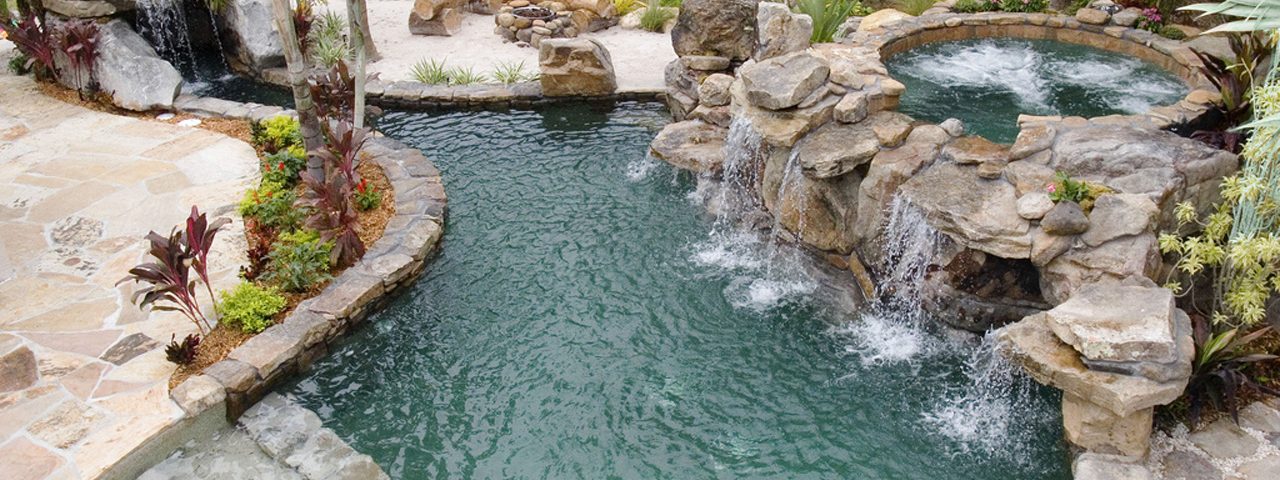This aerial photograph captures a beautifully designed, large backyard pool with an intricate stonework border. The pool, shaped partly by a semicircular stone wall, features an elevated area on the right that resembles a natural rock formation, enhancing the organic aesthetic of the scene. This elevated area houses a jacuzzi, which sits above the main body of the pool, allowing water to cascade down the stacked boulders, creating multiple picturesque waterfalls that pour into the pool below. Swimmers can enjoy the flow of water as it pools beneath these falls. Surrounding the pool, there is a stone pathway and well-manicured landscaping with various plants, adding to the natural ambiance. To the left of the pool, a patch of dirt supports several trees, contributing to the lush, green backdrop. The overall effect is a harmonious blend of natural and manufactured elements, resembling a serene oasis.